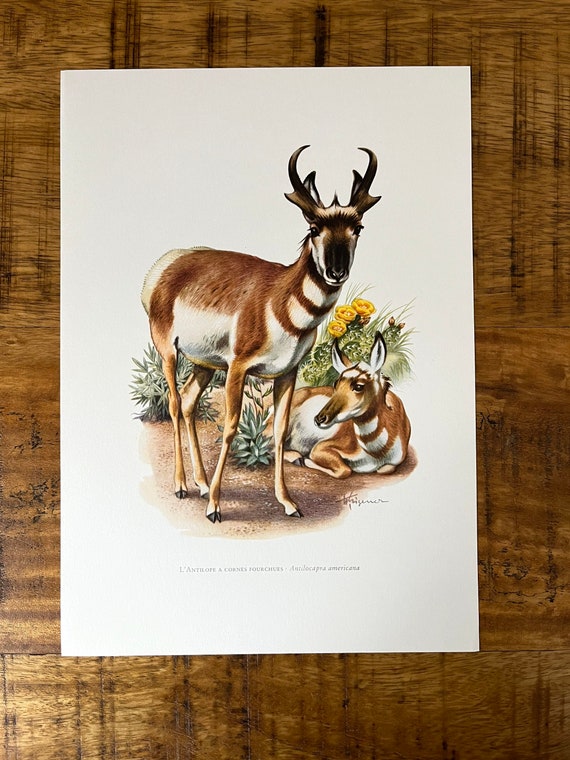This image captures a drawing placed on a wooden floor, viewed directly from above. The drawing, set against a white background, prominently features two deer-like animals. Centered in the image is a standing deer with its body turned slightly to one side. Its head, a mix of dark and light brown, faces to the right, revealing two antlers that curve inward. The deer's back and neck display alternating brown and white stripes, while its belly is white and its tail is white. Its legs are a lighter shade of brown. Lying on the ground to the lower right of the standing deer is another deer of similar coloring, but with white ears and no antlers. The scene includes sparse details of green grass, three yellow flowers next to the standing deer's neck, a green plant growing between its legs, and a brown ground beneath them. The detailed rendering of the animals, with features such as a flattened face in the standing deer and the absence of antlers in the reclining deer, suggests careful attention to contrasting textures and patterns within the drawing.